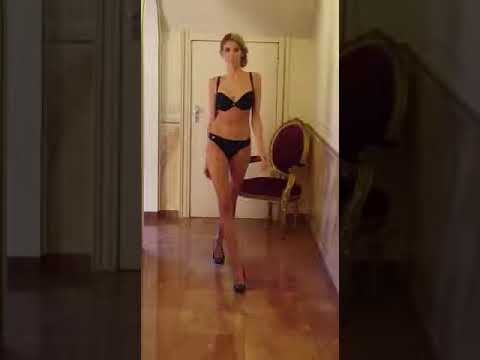This photograph captures an indoor scene featuring a tall, thin, blonde woman with shoulder-length hair walking gracefully across a glossy, wooden hardwood floor. She is dressed in a black bikini, comprising a bra-style top and regular bottoms with a white spot on the right hip, paired with black spiked high-heeled shoes. The woman, who has long legs and fair skin, maintains a neutral expression as she moves. Dominating the background is an antique, Victorian-era chair with black upholstery and a gold frame, positioned against a backdrop that includes a white door and drapes. The lighting, sourced from the left side of the image, suggests natural daylight. This image forms a central panel flanked by two blurred, black-out panels on either side, enhancing the focus on the woman and the elegant, vintage chair behind her.